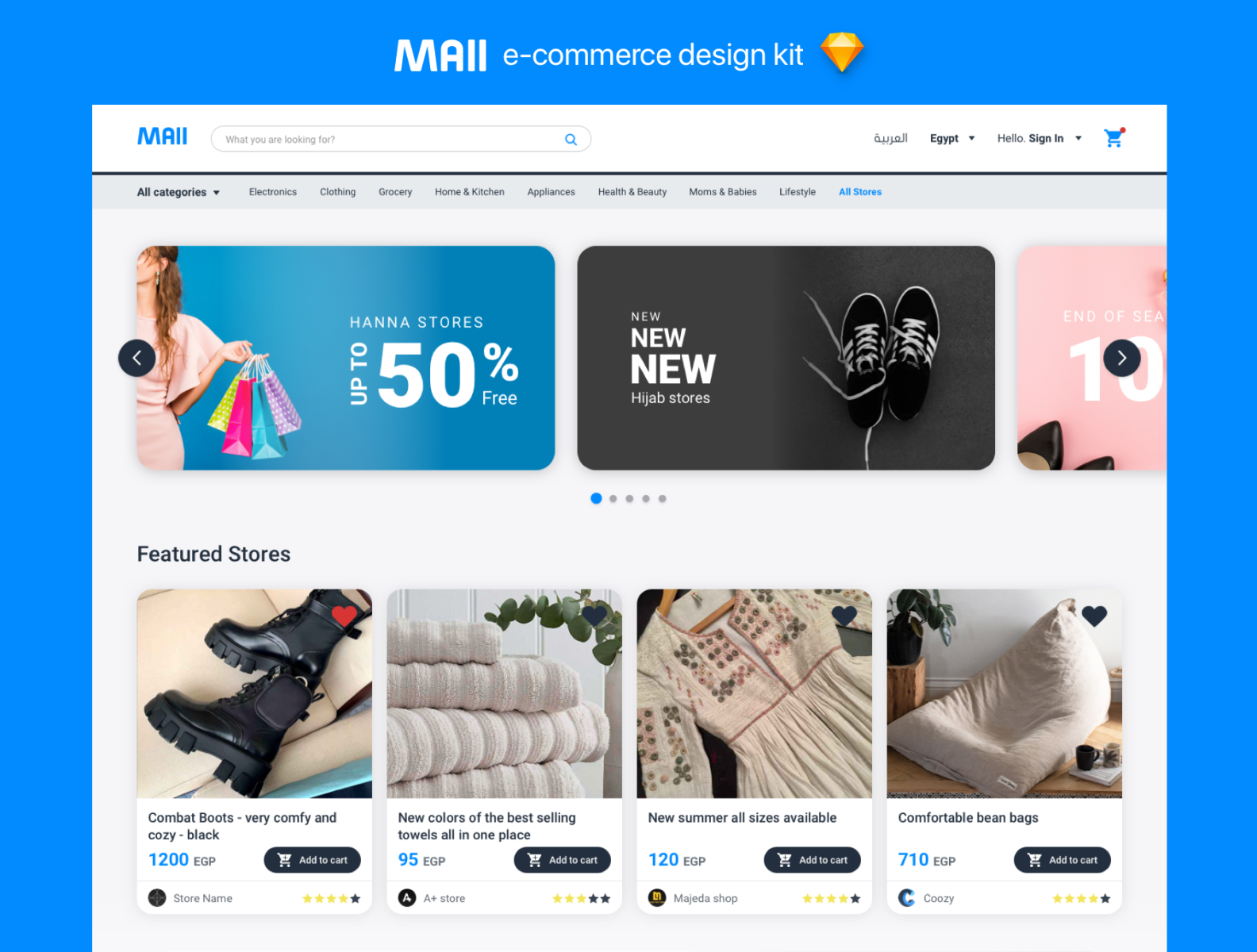This detailed caption describes a screenshot of a website with emphasis on its layout, design, and specific content elements:

The screenshot captures a web page featuring a blue border that frames the left, top, and right sides of the display. Centered is a white vertical rectangular area that includes various navigational and content elements. At the top middle within the blue border, the word "Mall" is prominently displayed in bold white letters. Adjacent to this, in regular white font, is the phrase "E-commerce Design Kit," complemented by an icon of a yellow diamond located to the right.

Beneath this title section, again in bold blue letters, the word "Mall" reappears, followed by a search bar to the right. Continuing rightwards, there's a word too blurred to identify, and further along, the word "Egypt" appears in dark gray with a downward-facing arrow next to it. Beyond this, the site offers a "Hello, Sign In" option, also in dark gray with another downward arrow. To the far right, a blue shopping cart icon is located, marked with a red circle at the top-right corner.

Below the navigation bar are category buttons, starting with "All Categories," which is highlighted in black and accompanied by a downward-facing arrow. To the right, additional categories are listed: "Electronics," "Clothing," "Grocery," "Kitchen Appliances," and "Health and Beauty." The last two categories are too blurry to decipher, and to the far right, a blue-highlighted category labeled "All something" is visible, though the second word is unclear.

Further down the page, two thumbnail images are displayed. The first thumbnail, with a blue background, features a pale-skinned woman holding four colorful shopping bags, with a left-facing arrow on the left side of the image. To its right, another thumbnail with a dark gray background contains the word "New" repeated thrice, increasing in size from top to bottom ("new, new, NEW"). Beneath this text, the words "Hijab Stores" appear in small gray font. The right side of this image showcases black sneakers with white shoelaces.

Finally, on the extreme right, a partly cut-off image with a pink background displays the number "10" in large white font across the middle, and at the bottom left corner, the tips of high-heeled shoes are visible.